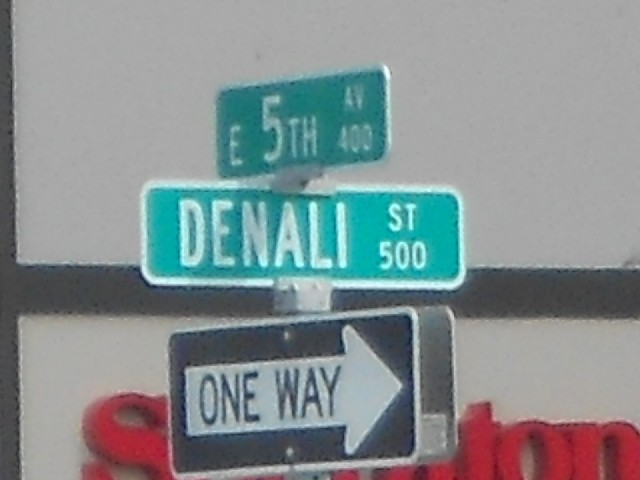In the image, three distinct highway signs are prominently displayed against an urban backdrop. The top sign, a green rectangular plaque, reads "East 5th Avenue 400" in bold, white text, indicating the street name and direction. Below it, the second sign marks "Denali Street 500," with "DENALI" written in large, white, capital letters, ensuring visibility. The bottom sign, a black-and-white one-way indicator, directs traffic to the right. In the background, a business establishment is visible, characterized by its red lettering.